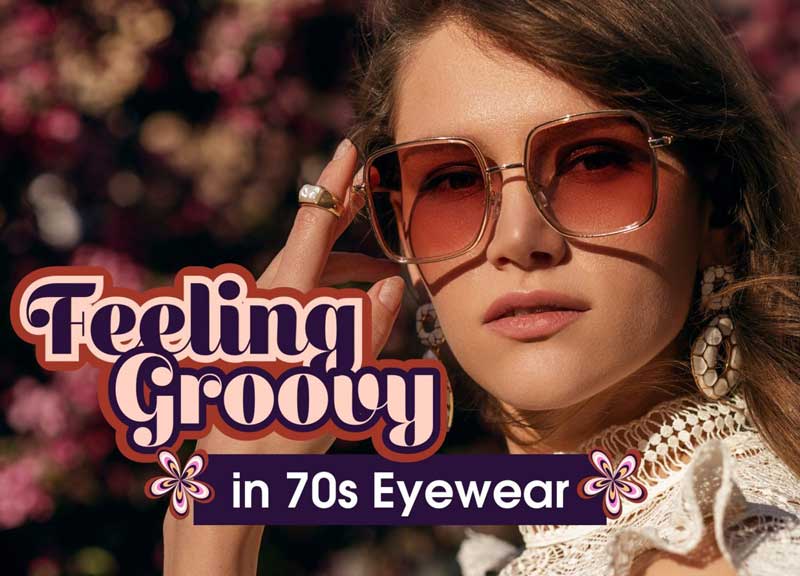This vintage-inspired advertisement for eyewear captures a woman set against a blurry, flower-filled background, exuding a nostalgic 70s vibe. The focal point is a woman with long, straight brown hair, styled in a lacy top with a prominent high collar. She accessorizes with chunky, circular white earrings and a unique knuckle ring on her index finger. Her standout piece is a pair of oversized, square-shaped red sunglasses. With her hand partially raised, she confidently faces the camera, emitting a sense of effortless cool. Bold text adjacent to her reads, "Feeling Groovy in 70s Eyewear," perfectly encapsulating the retro theme.